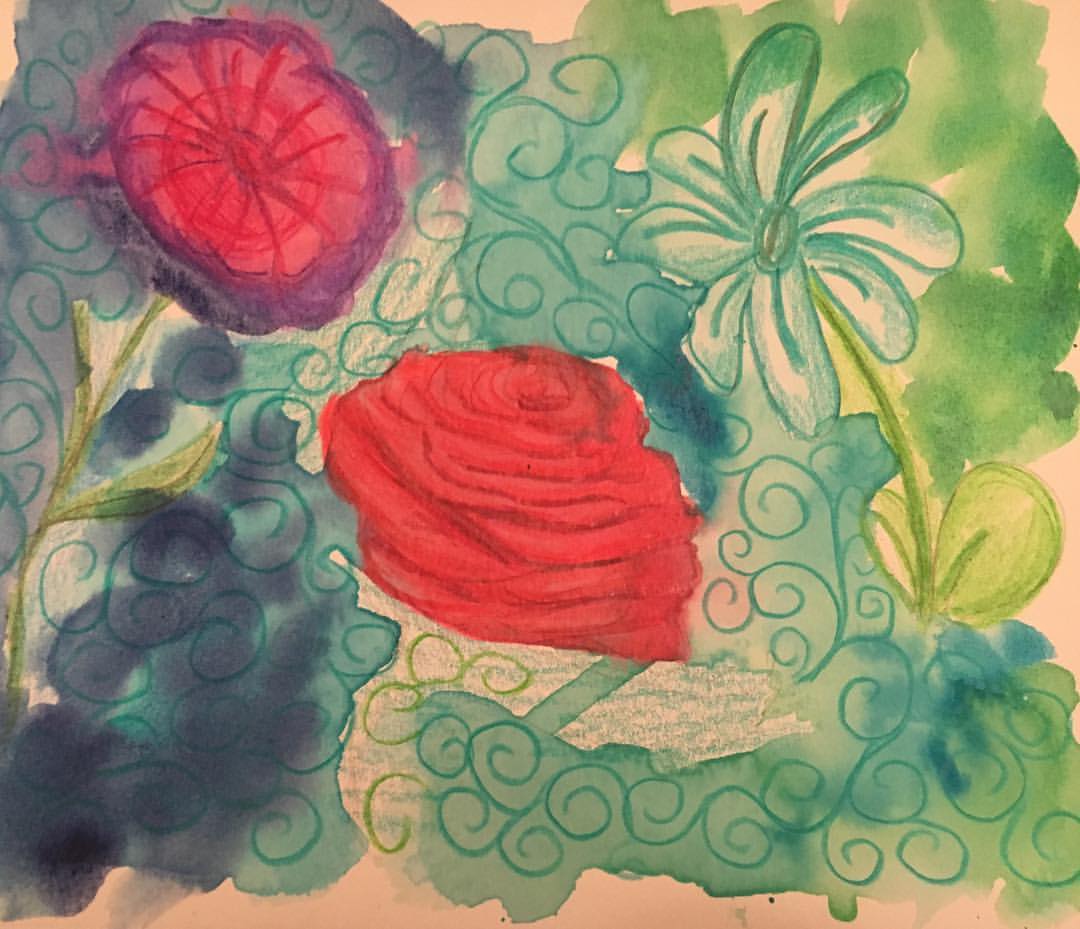This painting exhibits a vibrant watercolor composition featuring three distinct flowers set against an expressive background. In the top left corner, a striking flower portrays a captivating blend of red hues with purple accents along its outer edges. It is anchored by a long stem adorned with two delicate leaves. On the right side, a complementary blue flower mirrors the simplistic charm of a quintessentially drawn blossom, also supported by a pair of leaves. Dominating the bottom center, a rich, red rose captures attention with its classic elegance. Surrounding these floral elements, a dynamic array of swirling patterns infuses the scene with movement, created with a spectrum of blues and greens—ranging from dark blue and indigo to light blue and varying shades of green. The overall effect is a mesmerizing harmony of color and form, vividly rendered in watercolor, bringing the flowers and their intricate surroundings to life.